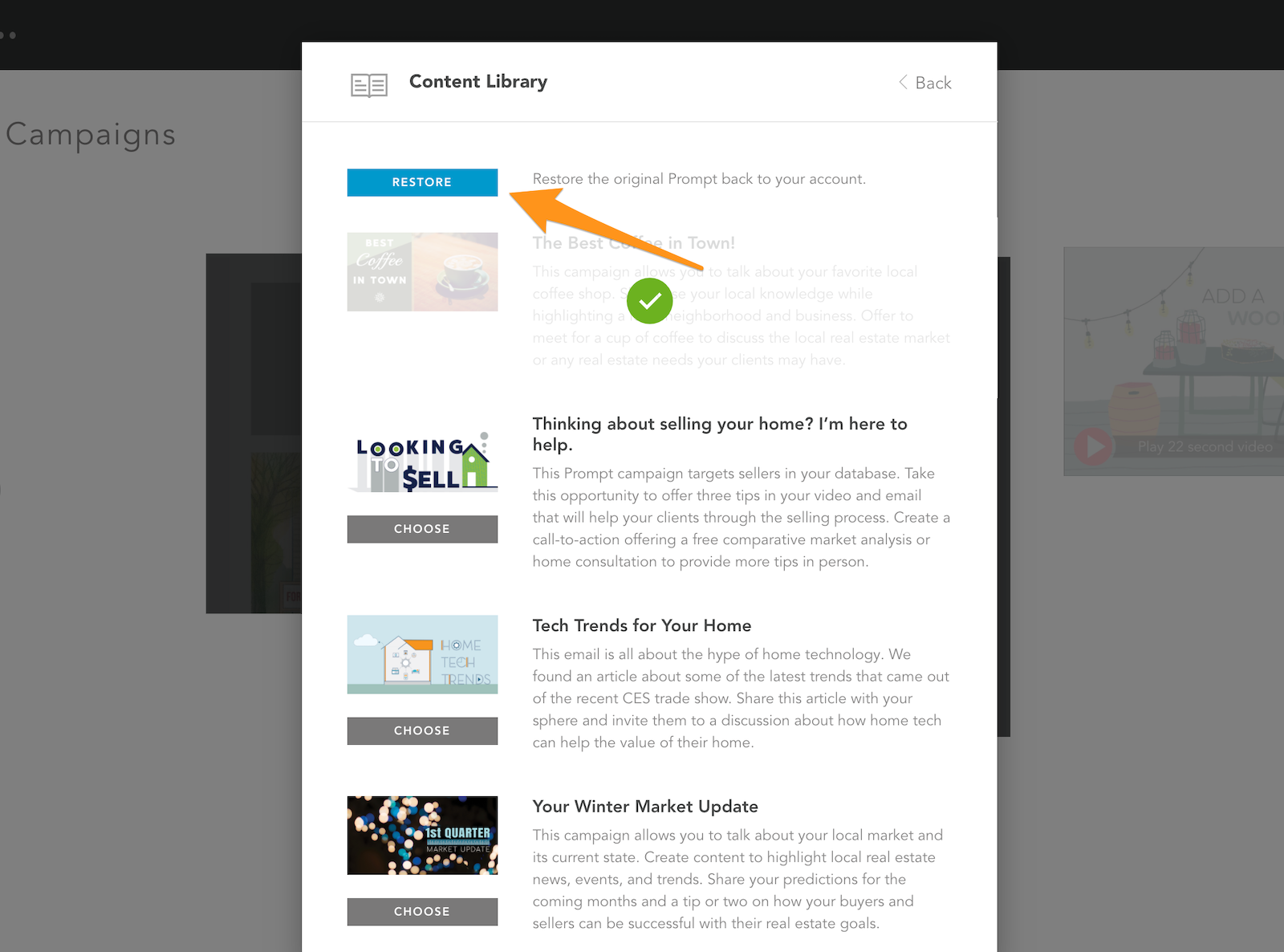The image displays a white pop-up page with detailed elements related to content and campaigns. In the upper left-hand corner, the pop-up is labeled "Content Library" in dark gray text. On the upper right side, there is a light gray "Back" button, accompanied by an arrow pointing to the left. A thin gray line runs horizontally across the page.

Beneath this line, a blue rectangle features the word "Restore" in bold white letters. An orange arrow points to this blue rectangle. Following this, in gray text, it reads: "Restore the original prop back to the account."

Further down, a promotional campaign titled "The Best Coffee in Town" is described. This campaign allows users to discuss their favorite coffee shop and includes a green circle with a white checkmark, although the associated text is partially obscured. The campaign encourages engagement with local knowledge and the local community, suggesting meeting clients for coffee to discuss the real estate market or other needs.

The subsequent section features a blue heading reading "Looking to Sell," followed by a gray box with white text that states: "Thinking about selling your home? I'm here to help."

Another category titled "Home Tech Trends" appears next, with a gray box discussing technology trends for the home.

Below, another section is titled "First Quarter Market Update" in blue text, followed by a gray box that mentions the winter market update.

The background varies, with the top part in black and the remainder in white, predominantly on the left-hand side. In the upper left part of the pop-up, the word "Campaigns" appears in gray text. On the right side, partially cut off, there is the phrase "Add a W-O-O," but it is not fully visible.

This detailed caption provides a thorough description of the elements and content displayed within the pop-up page.